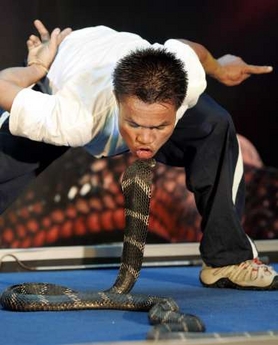In this close-up image, a daring snake charmer is seen leaning forward to kiss the head of a striking king cobra. The man, wearing a white t-shirt, black track pants with a white stripe down the side, and brown shoes, dominates the center of the frame. He has short, spiky hair and his hands are positioned uniquely: his left arm extends sideways with his index finger pointing out, while his right arm bends behind his back, extending his middle finger. The cobra, a formidable black serpent with white or gray stripes, has its head puffed and poised in a striking position, facing the charmer’s puckered lips almost in contact. The scene unfolds on a blue carpet-like flooring, with a white barrier visible in the background, and the man appears undeterred by the cobra’s threat. The setting seems to be indoors, possibly on a stage, intensifying the audacious nature of this mesmerizing encounter.